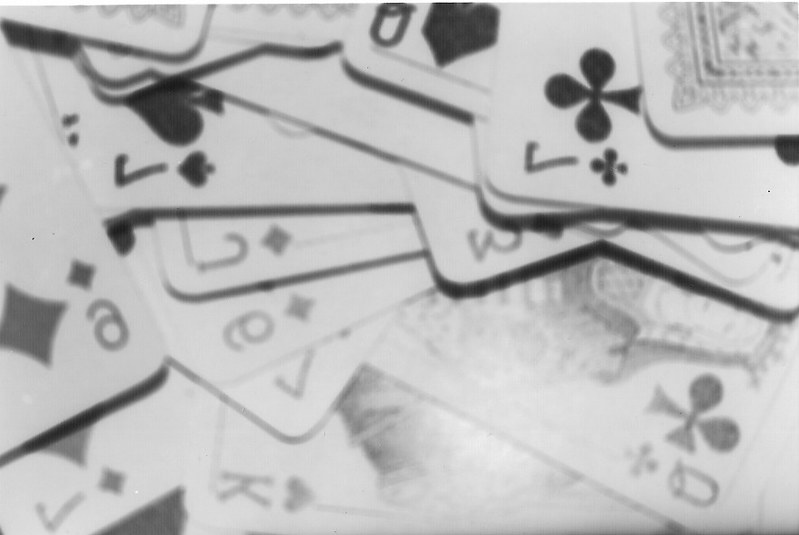A slightly out-of-focus black-and-white indoor photograph capturing an overhead view of a cluttered pile of playing cards, primarily arranged diagonally from left to right with significant overlapping. The image showcases 14 face-up cards interspersed with a few face-down cards that reveal the patterned backs.

From left to right and noting notable overlaps:
In the lower-left corner, the Seven of Diamonds is slightly over the Nine of Diamonds. To the right at the bottom, the King of Hearts is partly covered by the Seven of Diamonds. Further overlapping cards include the Six of Diamonds, Jack of Diamonds, and the Seven of Spades. A portion of the Three of Diamonds is peeking out from the right of the center of the pile. In the upper center, a partly obscured Queen of Spades is visible. The lower right corner reveals most of the Queen of Clubs, while the upper right corner shows the Seven of Clubs.

The photograph also exhibits a light glare concentrated in the lower right portion, further emphasizing the black-and-white aesthetic and the somewhat jumbled arrangement of the cards. Other than the card numbers and suits, there is no additional text or print visible within the image.